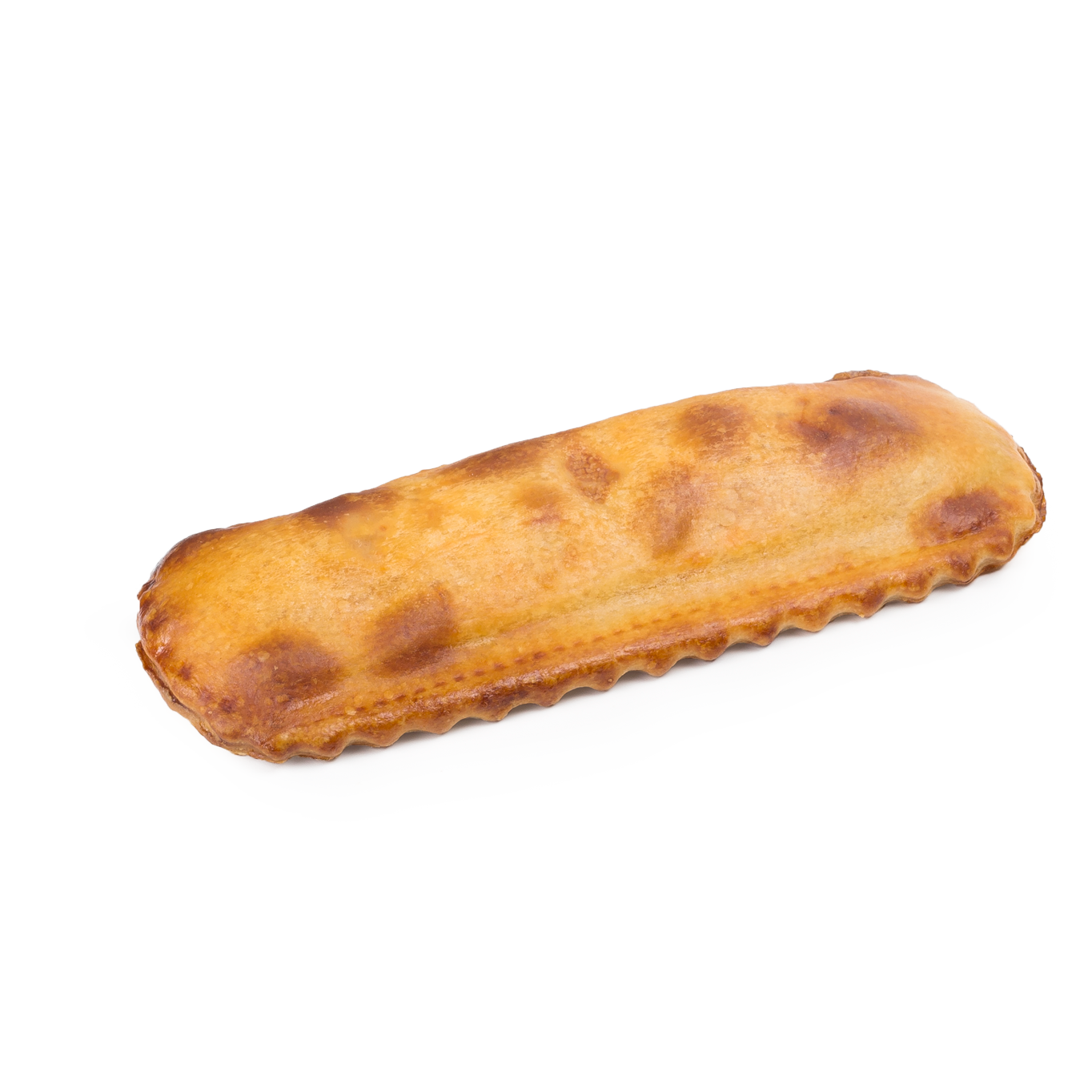The professional photo, captured against a crisp, solid white backdrop, showcases a well-lit and perfectly in-focus rectangular pastry. The pastry, likely a type of puffed pastry akin to those found in cafes, is a warm light brown color with irregular splotches of darker, almost burnt brown. The edges are meticulously crimped, suggesting an enclosed filling, potentially applied by the tines of a fork or a specialized crimping tool. This sealing method hints at a variety of possible fillings, such as meat, cheese, chocolate, or fruit. The pastry's shape is slightly elongated with rounded ends, and while predominantly flat, the bottom features gentle waves. This type of pastry is not only popular in the United States and England but also resembles savory pastries from Jamaica. The image is devoid of any text, allowing the focus to remain entirely on the detailed texture and form of the pastry.